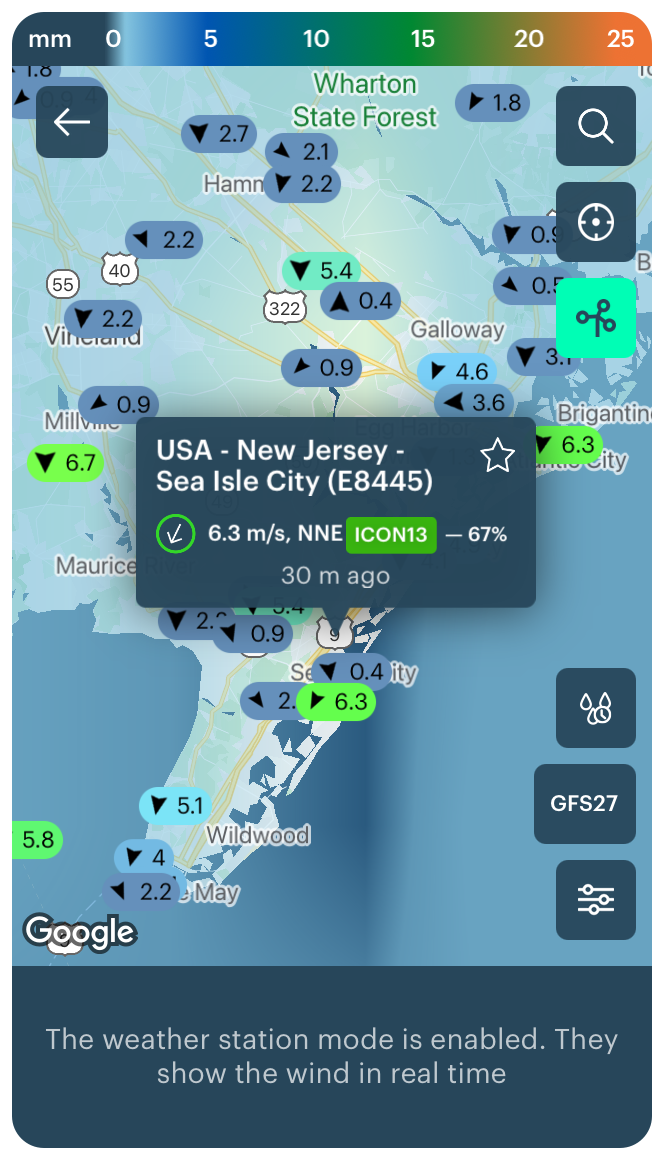This detailed map illustrates various locations within the United States, specifically pinpointing Galloway, New Jersey, among other areas including Queensland, Millville, Maurice, May, Wildwood, and Bregantown. Also marked is Sea Isle City. Data icons suggest dynamic elements such as movement at 6.3 miles per second in the north-northeast direction, and an indicator showing 67% that updates every 30 minutes. Below the map, the Weather Station Mode is activated, providing real-time wind conditions for the area.